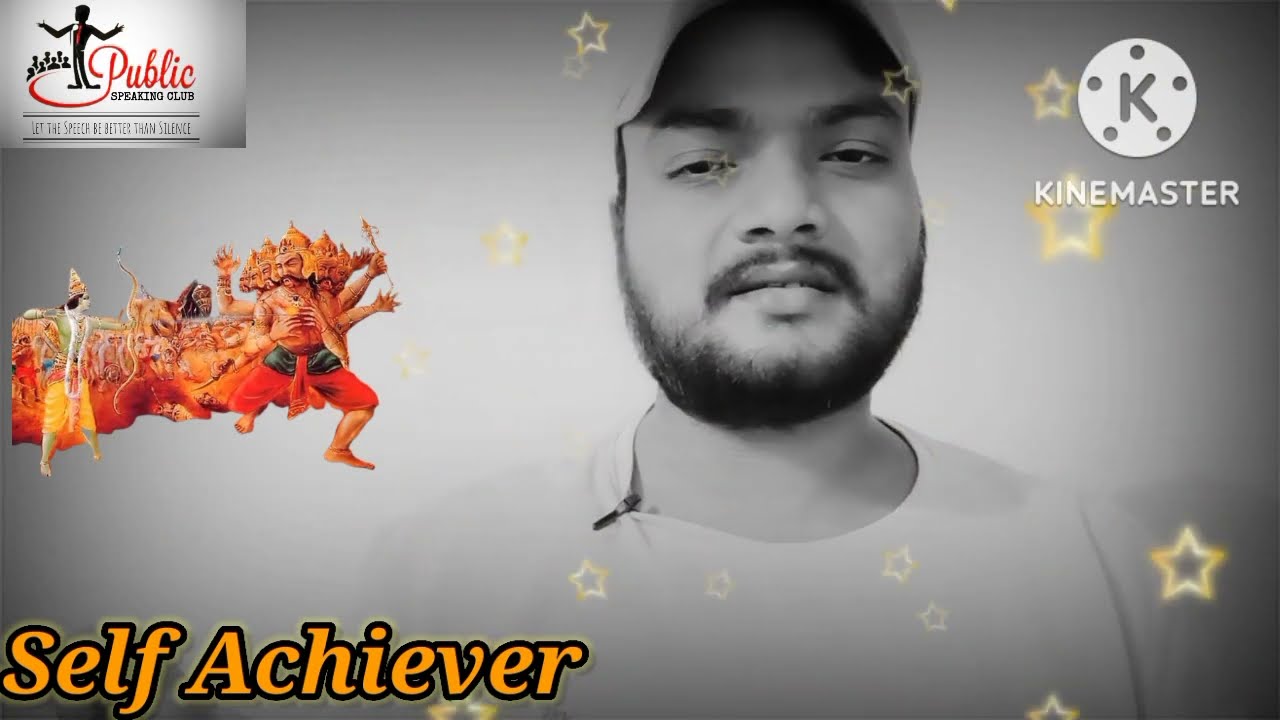The black and white screenshot portrays a man of South Asian descent with distinctive facial features, including a thick black beard, mustache, and bushy eyebrows. He is wearing a white baseball cap and a white crew neck t-shirt with a black microphone attached to the collar. The man's face is slightly blurred at the top, and he appears to be looking downward with his mouth slightly open.

The image contains several text elements and logos. In the upper right-hand corner, there is a white circle containing a black letter 'K' surrounded by five black circles, with the word "KindMaster" written below it. This logo is associated with a video editing application. Golden stars are scattered across the image.

In the upper left-hand corner, a black-and-red logo depicts a human figure with raised arms next to the text, "Public Speaking Club." Below this logo is an elaborate depiction of South Asian cultural figures, featuring a man performing a dragon dance and goddesses adorned in red and orange costumes with ornate gold headpieces, holding gold rods and dancing.

Finally, in the lower left-hand corner, yellow-orange text with a black outline reads "SELF-ACHIEVER," further emphasizing the inspirational tone of the image.